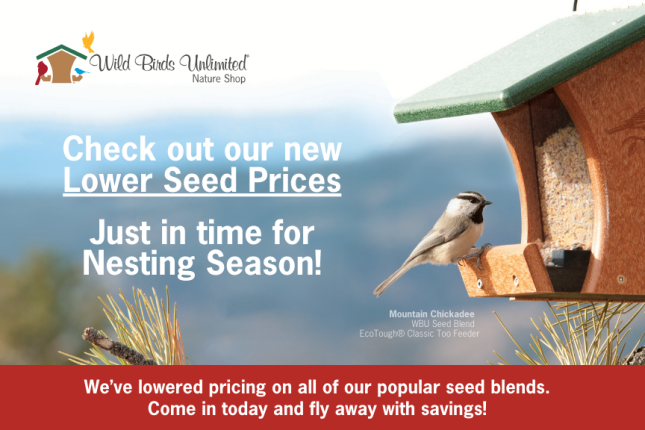The advertisement image for Wild Birds Unlimited Nature Shop prominently features a beautifully detailed scene emphasizing the store’s new pricing on bird seed. At the very top left, the logo "Wild Birds Unlimited" is displayed. Below, bold white text announces, "Check out our new lower seed prices just in time for the nesting season." Adjacent to the text, a Mountain Chickadee—a small bird with a white head, grayish body, and a small beak—is perched on a wooden bird feeder with a green roof. The feeder is filled almost to the brim with bird seed, framed against a blurred mountainous background that includes tree branches. At the bottom of the advertisement, additional text states, "We've lowered pricing on all of our popular seed blends. Come in today and fly away with savings." The vibrant colors in the image include various shades of blue, white, green, brown, and gray, which help highlight the natural beauty and allure of bird watching.